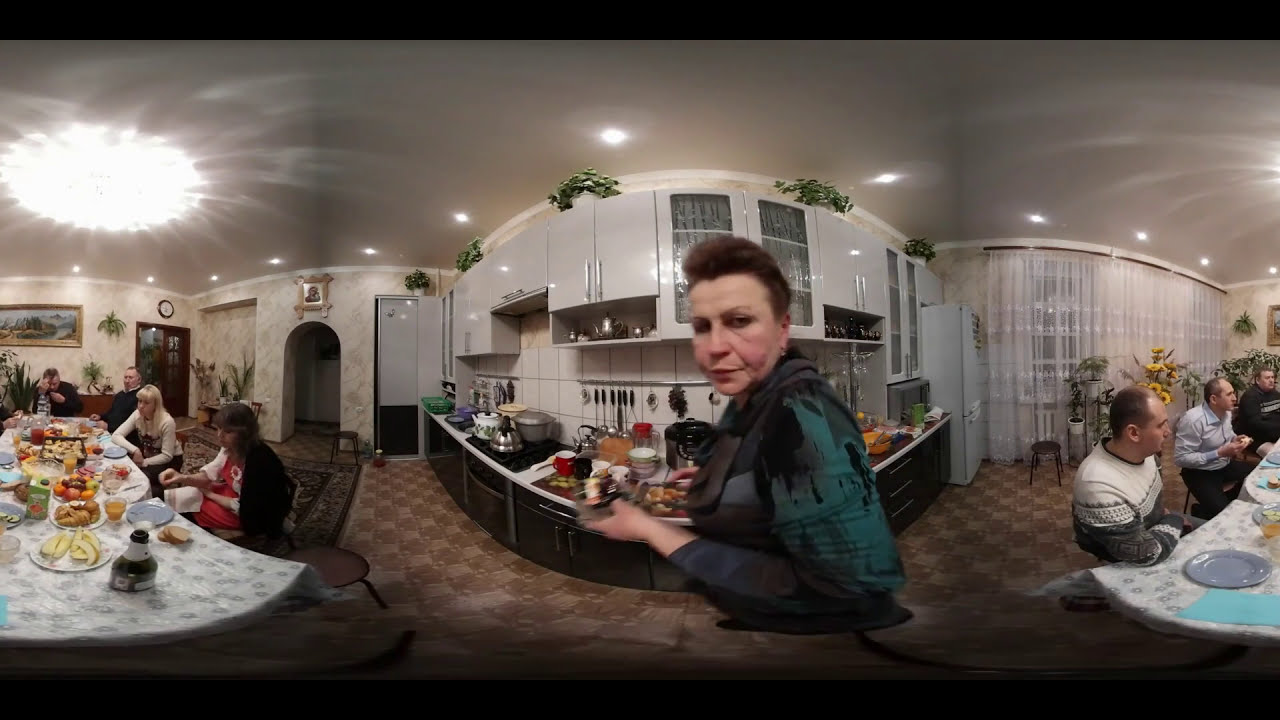In this image, people are seated at tables enjoying a meal, seemingly in a cozy, restaurant-like setting. The room features a brown floor and has a harmonious color palette dominated by whites and grays, including white kitchen cabinets, a white ceiling, and sheer white draperies. The tables are set with a variety of colorful dishes, featuring reds, yellows, and greens. Prominently, a woman stands at the center, possibly a hostess or waitress, wearing a green long-sleeved top with her short brown hair pulled back, showcasing her rosy, jowly cheeks. She holds something in her hand and stands against a backdrop of a bustling kitchen area crowded with white metallic cupboards and various kitchen gadgets. On top of the cabinets, there are house plants adding a touch of green to the scene. The back wall is adorned with paintings in gold frames and has some plants, both green and yellow. 

To the right side of the image, three men are seated at a table, one in a blue business shirt, another in a sweater, and the third person who is less discernible. To the left, another table is visible with women seated, including one in a white sweater and another in a red dress. Above this table hangs a bright, circular chandelier. The atmosphere is lively with people engaging in conversation and waiting for their food, offering a warm and social dining environment.